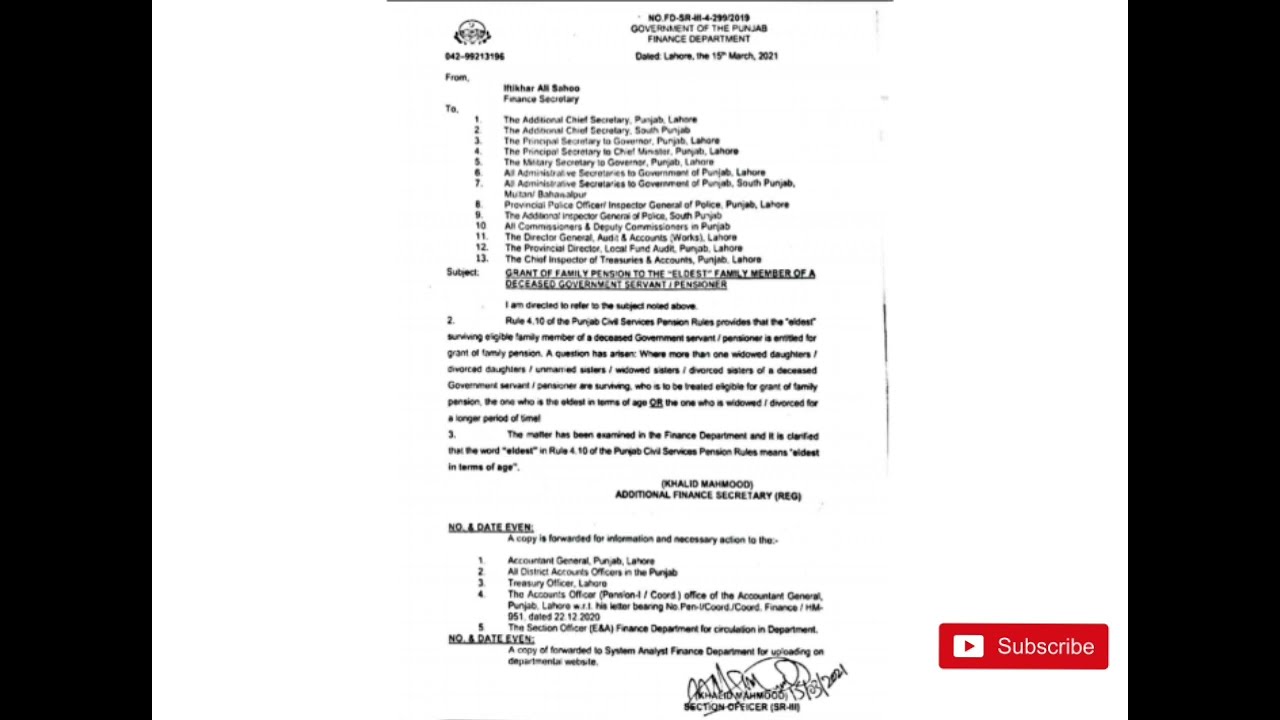The image is a screen grab from a YouTube video, featuring a black-and-white scanned or photocopied document on a wide white rectangle, flanked by black bars on the sides. The document, from the Government of the Punjab Finance Department, is dated 15th March 2021. It addresses the subject of granting a family pension to the eldest family member of a deceased government servant or pensioner. The upper right section of the document includes a grid and mentions the Finance Secretary. The document is mainly composed of a 13-point bullet list detailing director-general positions, names, and geographical locations. Below the list are a couple of paragraphs followed by additional numbered sentences from 1 to 5. At the bottom of the document, there is a visible signature next to the title "Section Officer" with some text in parentheses. In the lower right corner of the image is a red YouTube "Subscribe" button with white text, indicating its origin from a video.